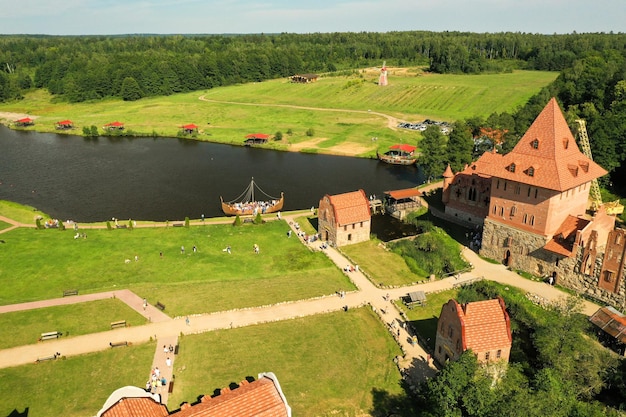This panoramic daytime photograph, likely taken from a drone or a helicopter, captures a serene, pastoral landscape marked by a patchwork of grasslands and a meandering river. Dominating the right-hand section of the image is a notable old, Renaissance or Gothic-style building with stone walls on the lower floors and wooden upper floors, topped with a red gable roof and adjacent to a ladder. This building is complemented by smaller structures of similar architecture—stone with red gable roofs—scattered about the scene, including one prominent building with off-white walls.

Paths traverse the scene, including a trident-shaped walkway in the left quadrant of the field, leading to various stone pathways where small figures can be seen strolling. In the mid-ground, a river flows, grey in color, with a wooden, single-mast ship resembling a Viking vessel docked along its bank. This river is lined with green grass and stone pathways.

Beyond the river, on its opposite bank, are numerous single-story houses with red gabled roofs, surrounded by lush green grasslands. Farther back, there's a windmill standing amid trees, indicating a possible rural Dutch setting. The backdrop features a dense forest and a sky that transitions from blue to white, enhancing the bucolic charm of this tranquil landscape.